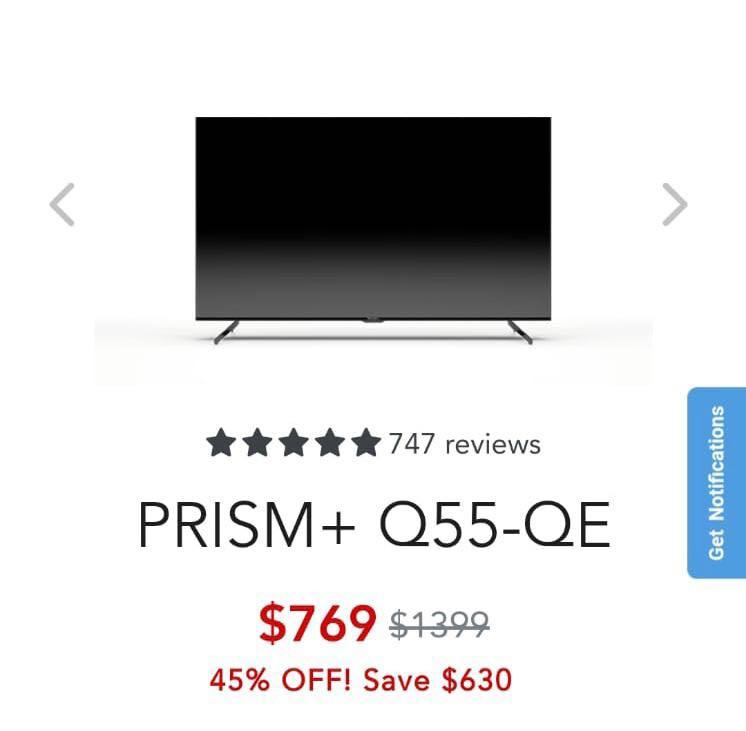This detailed image features a product for sale, specifically a PRISM+ Q55-QE television set. The TV is centrally positioned against a white background, showcasing its sleek design with a black screen turned off and small, sturdy black legs on either side at the bottom. Flanking the image are two gray arrows, one on the left pointing left and another on the right pointing right, likely for navigating through the product images.

Beneath the TV, there is a rating display showing five black solid stars, indicating positive customer feedback with "747 reviews" written next to it. On the far right, a vertical blue rectangle runs from bottom to top with the text "Get Notifications" oriented vertically.

Further details include the model name "PRISM+ Q55-QE" in large, bold, black capital letters. Directly below, the pricing is highlighted: a striking red dollar sign and price "$769," contrasted with a gray original price "$1399" that is struck through. Additionally, in bold red text, the image announces a "45% OFF" discount, emphasizing a savings of "$630."